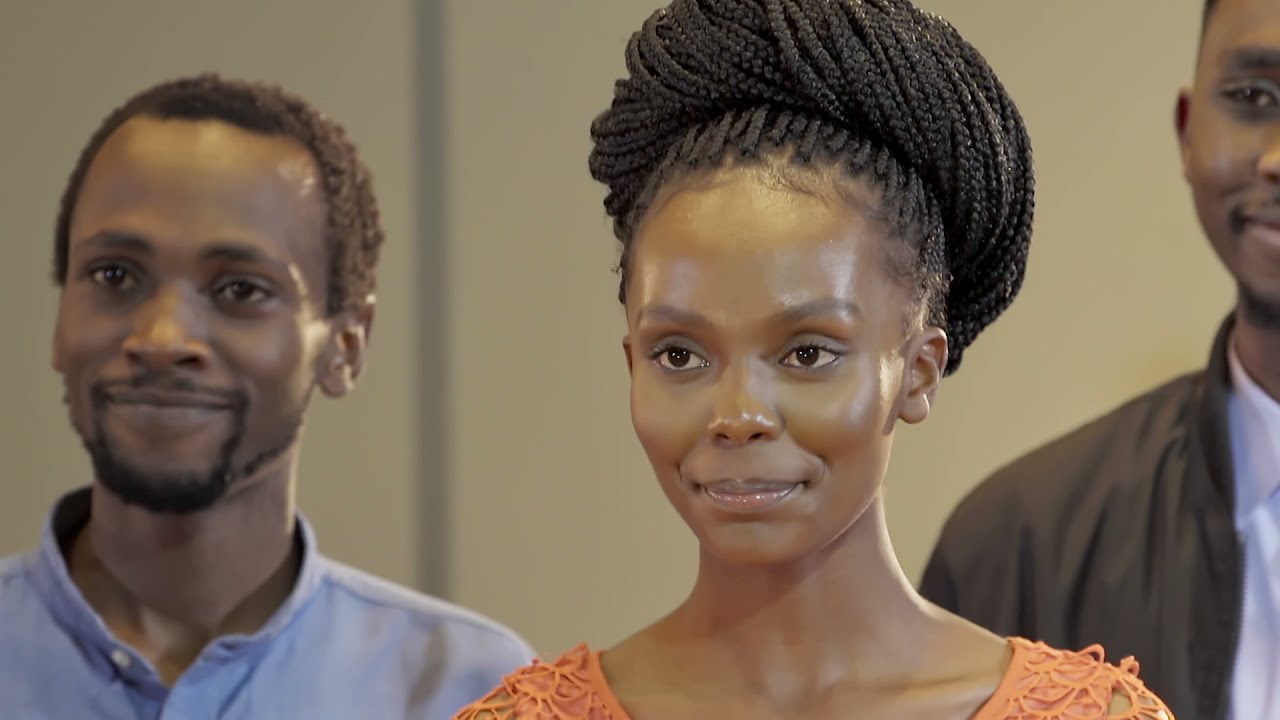In the center of the image, there is a Black woman with smooth, shiny skin and deep brown eyes, her face prominently positioned. Her hair is styled in cornrows gathered in a bun at the top of her head. She is wearing an orange shirt with a decorative, stringy leaf pattern, and her collarbone is visible. She appears to be looking off to the left side of the image with a serious expression. Flanking her are two smiling Black men from the shoulders up. To her left, a man with short, fluffy black hair, a thin mustache, and a goatee is dressed in a light blue button-up shirt with a collar. To her right, partially cut off from the frame, is another man in a black overcoat and white collared shirt. Both men are looking in the same direction as the woman, towards the left side of the image. The background features a plain tan wall, and the setting appears to be indoors, possibly in a public space. The image does not contain any visible text. The overall color palette includes shades of tan, brown, black, white, blue, orange, and gray.